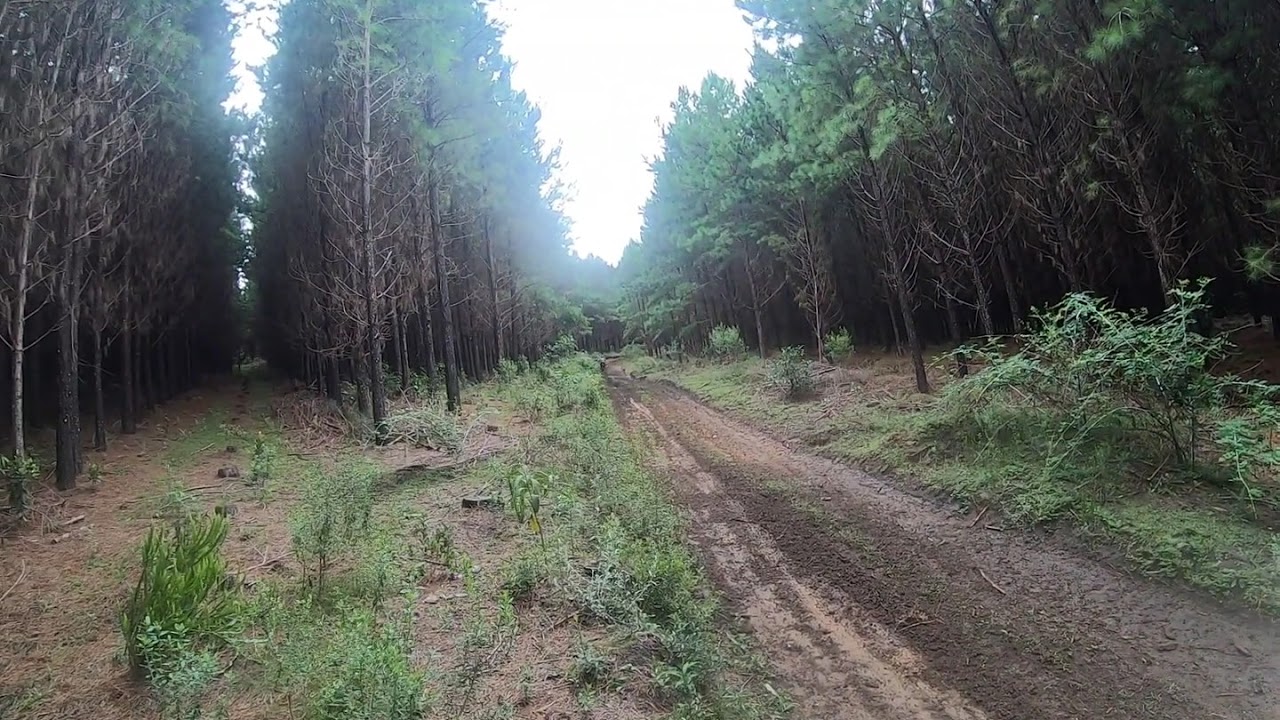The image captures a serene scene in a dense forest, dominated by an empty, narrow dirt road that winds from the lower right and tapers into the middle of the frame. Flanked by tall, dark trees—predominantly pines with their brown barks and sparse greenery—the road is enveloped in an atmosphere of seclusion and tranquility. On the right side, the ground is interspersed with brown dirt patches and overgrown bushes that almost encroach upon the road. The left side mirrors the dense, towering pines and patches of green foliage but is punctuated by another smaller path leading into a darker, more enclosed wooded area where the trees merge into a canopy, limiting the view of the sky. In contrast, the main road showcases glimpses of a bright, white sky that filters through the leafy curtain above, creating a stark yet welcoming brightness against the earthy and wooded landscape below.